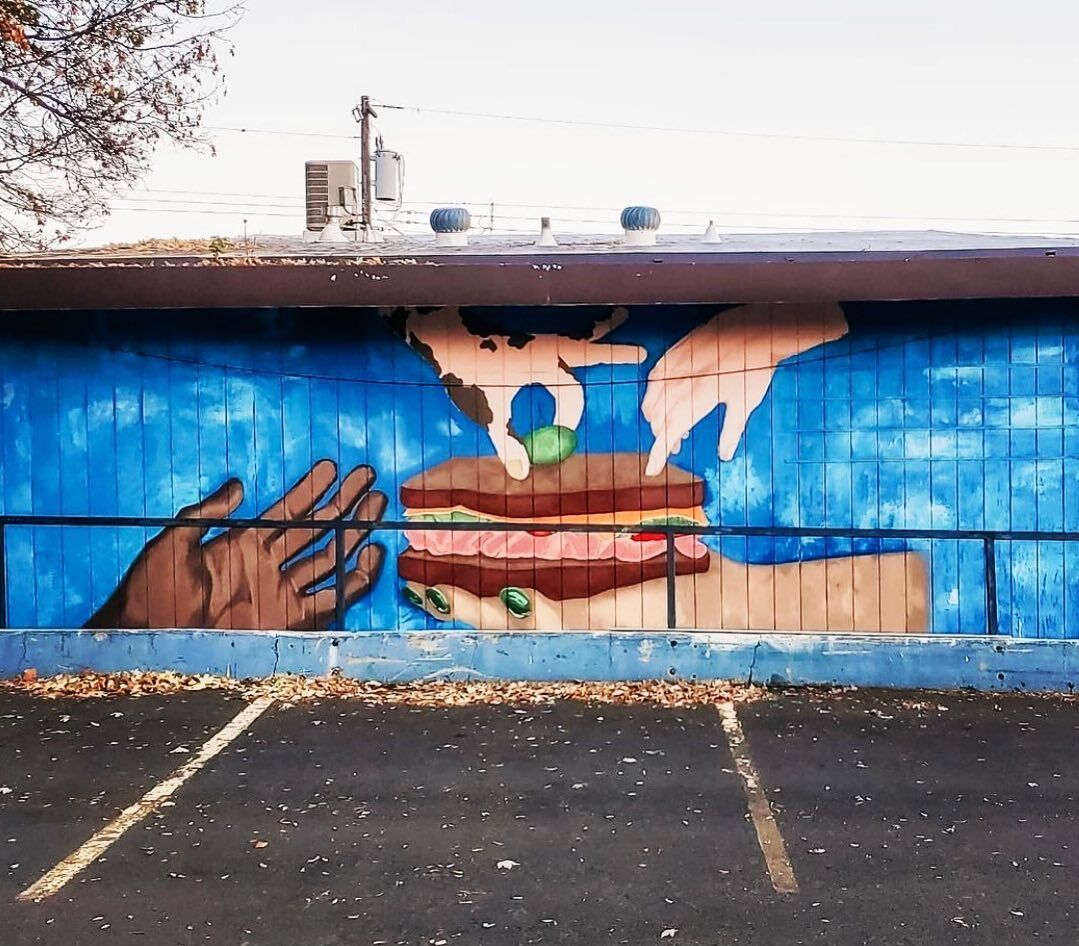This outdoor photograph captures a detailed view of the side of a fairly short building with a brown, leaf-covered roof. The building is constructed from long wooden panels, and a utility pole appears in the background beneath a clear gray sky. In front of the building, there's a parking lot where the lines marking the parking slots are beginning to fade, and autumn leaves are scattered, especially towards the end of the lot. A low ridge with a railing separates part of the parking lot from the building. Dominating the building's exterior is a vivid mural against a blue backdrop with white accents resembling the sky. The mural features a detailed depiction of multiple hands, each engaged in crafting a sandwich with brown bread, turkey, tomatoes, lettuce, cheese, and an olive on top. One hand, painted with green nail polish, holds the sandwich, while other hands are seen placing the toppings and reaching toward it. A hint of an autumn tree peeks in from the top left of the image.